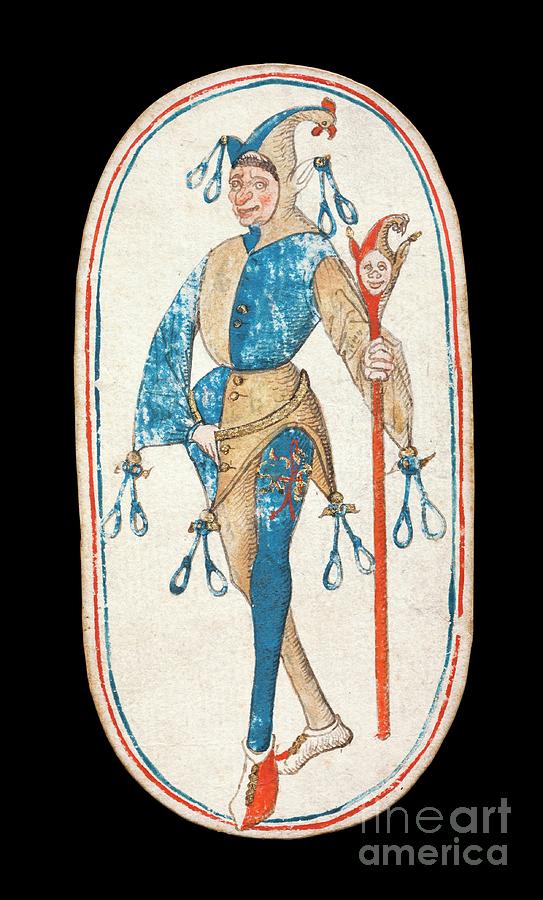This image from Fine Art America depicts a vividly detailed and whimsical portrait of a jester with a distinctly goblin-like face, set against a black background. The central figure is framed within a pill-shaped outline adorned with thin blue and red lines, encapsulating an off-white, cream-colored interior. The jester is dressed in a striking bicolored outfit: his left side features cream and orange hues, while his right side contrasts with blue. His attire is marked by alternating colors that extend from his hat to his shoes, with tassels dangling from various parts of his costume. 

He grips a red staff topped with a matching goblin-like head that also sports a similarly styled hat, seemingly mirroring his own. The jester's headgear is particularly elaborate, incorporating ear-like offshoots with dangling loops and culminating in a chicken head atop. His footwear reflects the same bicolored theme, with one shoe in orange and the other in white. The jester's face, framed by short brown hair, is turned to the left, displaying a mischievous smirk. Despite the medieval style of the illustration, some areas of the painting appear patchy, suggesting its age and historical charm. The bottom right corner bears a watermark reading "Fine Art America," identifying the image's source.